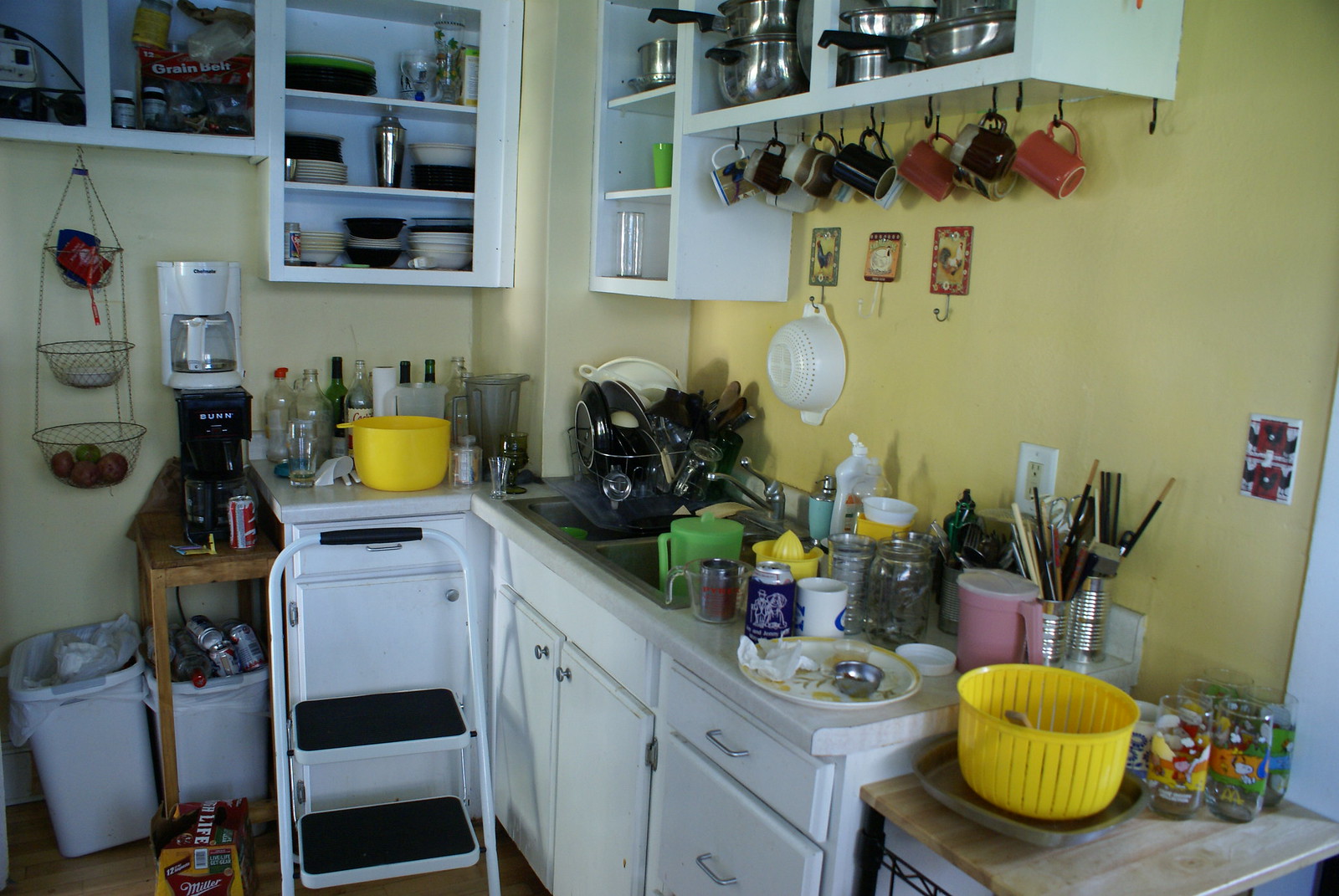The photograph showcases a busy and cluttered kitchen scene. Yellow walls frame the area, with numerous items filling every available space on the white shelves and countertops. At the top, around ten mugs are neatly hung on hooks. Various kitchen utensils, containers, and seasonings are scattered across the countertops, contributing to the disarray. A mini step ladder stands centered on the floor, presumably for accessing the higher shelves. Against one wall, a hanging bin filled with assorted fruits adds a touch of homeliness. Floral motifs and decorations embellish the light fixtures, adding a quaint charm to the space. The sink is piled with utensils and other kitchen items, indicating recent use. On the floor, there is a waste paper basket amid other miscellaneous objects. Several pots and pans are precariously stacked on top of the shelves, completing the picture of a kitchen bustling with activity and utility.